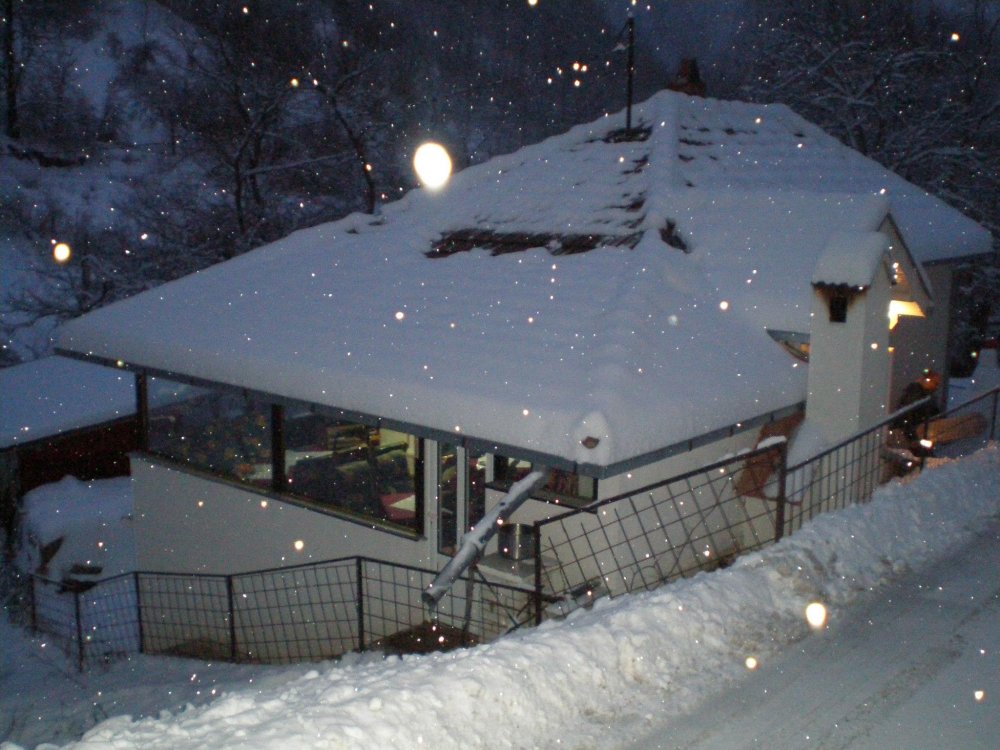This nighttime outdoor image captures a snow-covered house viewed from a higher vantage point, likely a road. The house, built on a hill, has a roof partially covered in snow with some dark patches revealing the tiles beneath. The scene is illuminated by a flashlight or camera flash, which highlights the falling snowflakes, giving them a star-like appearance. 

The upper part of the photo shows a snowy landscape with trees heavily laden with snow. The foreground reveals a flat, snow-covered area and a mound of snow descending toward the house, suggesting the photo was taken from an elevated road.

The house itself is white, with three horizontal windows on the visible left side, offering a glimpse of furniture inside, possibly a couch. It has a somewhat triangular rooftop due to the presence of a central chimney. On the less visible side, there’s a doorway with a light on. Surrounding the house is a dark-colored wire mesh fence with small square cutouts. The overall scene is serene and wintry, with the glow from the flash and inside lights contrasting against the dark, snowy night.